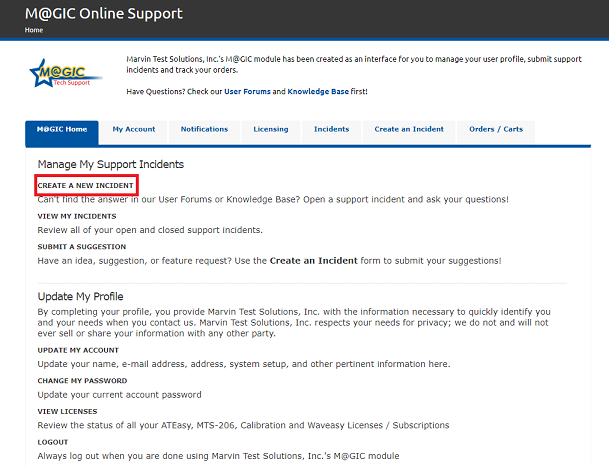The landing page for MAGIC Tech Support features a distinct and visually engaging logo. "MAGIC" is prominently displayed in black capital letters, with the "A" represented by an "@" symbol. Surrounding the "GIC" portion is an open blue star, which also underlines the word "MAGIC." The entire logo is highlighted with a yellow background, while the words "tech support" are positioned beneath the blue line in small red text.

A black banner spans the top of the screen. On its left side, "MAGIC Online Support" is written in white text, with "Home" in smaller white text directly below it. The remaining page is set against a white background.

Below the black ribbon, the MAGIC logo is aligned to the left. To its right, tiny navy blue text states, "Marvin Test Solution Incorporated's MAGIC module has been created as an interface for you to manage your user profile, submit support incidents, and track your orders." Below this, bold and bright text urges users, "Have questions? Check our user forums and knowledge base first!" The phrase "User forums and knowledge base" is in bright blue.

A series of horizontal tabs is displayed beneath the text, featuring options for navigating the site: MAGIC Home, My Account, Notifications, Licensing, Incidents, Create an Incident, and Order/Carts. These tabs rest on a light gray background with navy blue text, except for the MAGIC Home tab, which is highlighted in navy blue. A dark blue line runs underneath the unselected gray tabs.

Further down, black text reads "Manage My Support Incidents" followed by "Create a New Incident" in tiny capital letters, encased in a red box. The subsequent sections of the profile are dedicated to performing various activities such as managing support incidents, updating profiles, and other user-specific tasks.